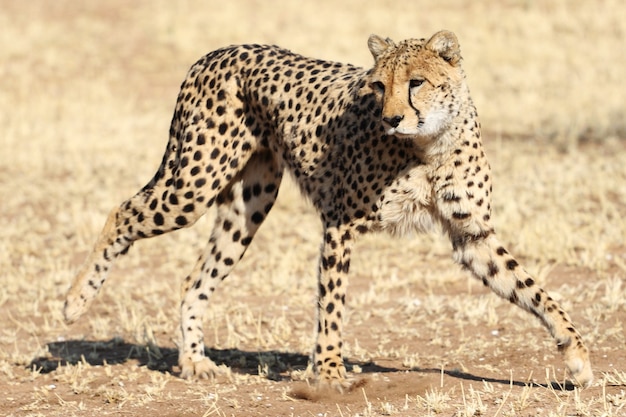This color photograph depicts a cheetah walking in the wild, amidst a dry and barren landscape. The cheetah, predominantly light brown with a darker hue on the top of its head, features iconic black spots covering its body. Black tear-like streaks extend from the inner corners of its dark eyes down to either side of its snout. Its nose is black, and the inside of its ears and the area below its chin are primarily white. The cheetah's large paws, some showing visible claws, traverse a field of dry, tan-colored grass interspersed with brown dirt, gravel, and sections of burnt grass and weeds. The background is slightly blurred, emphasizing the arid setting and the majestic animal as the focal point.